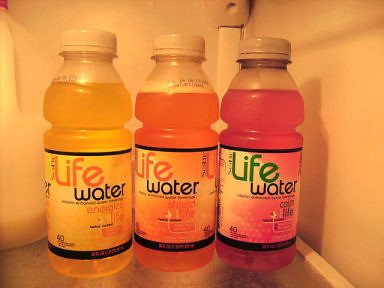The image showcases a warmly lit scene dominated by a yellow-orange hue. It features three Life Water sports drink bottles arranged in a row. The bottle on the left contains a yellow liquid, the middle bottle has an orange liquid, and the one on the right contains a red liquid. Behind the leftmost bottle, a gallon jug of milk is partially visible, with only half of it in the frame. The bottles are placed on a plexiglass shelf, and the white walls in the background suggest that the bottles are situated inside a refrigerator. The overall lighting and tone contribute to a cozy, inviting ambiance for the beverages.